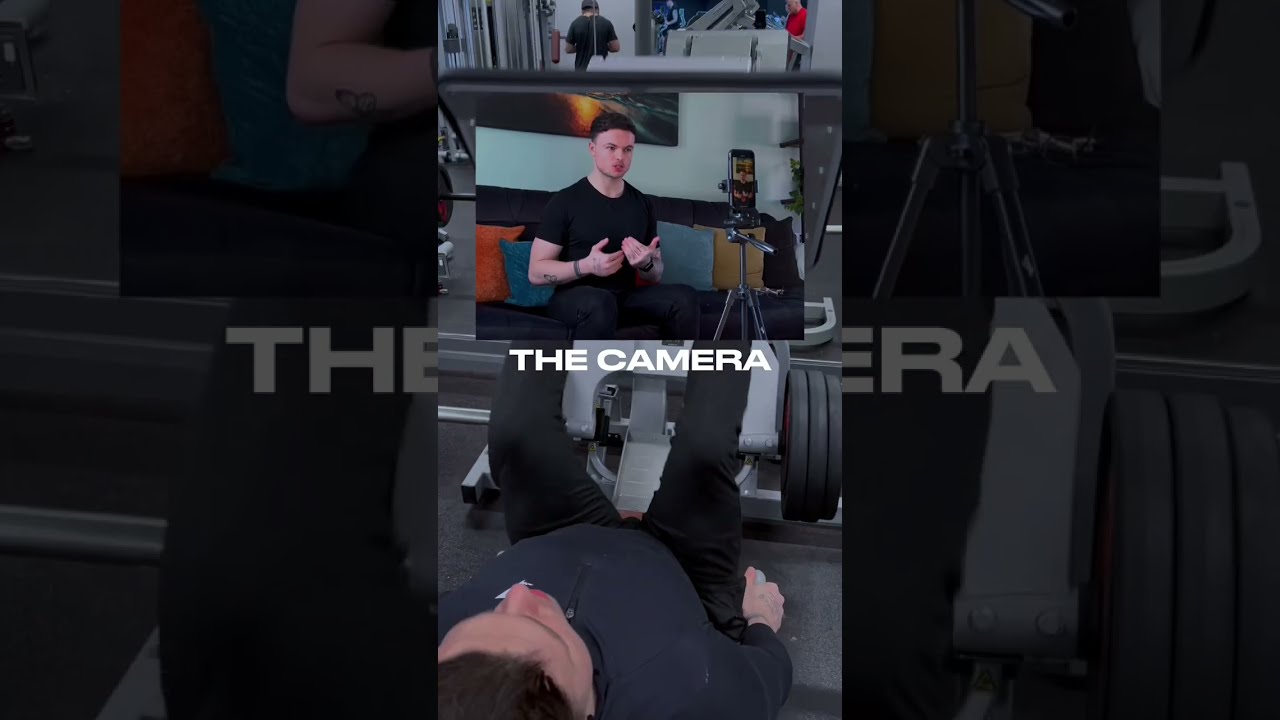The image features two layers, with a central inset picture within a dimly lit, zoomed-out gym backdrop. In the inner picture, a man, dressed in a black short-sleeve shirt and black pants, is seated on a black couch against a colorful array of pillows—orange, teal, and gold. He appears to be recording a video on his smartphone mounted on a tripod. Text in white capital letters reads "THE CAMERA" directly below him. Above the inner picture, in the gym background, the same man, identifiable by his short black hair and attire, is seen lying down, engaging in an exercise on a silver leg press machine, with black weights visible. His legs are raised, emphasizing his workout. The amalgamation of these visual elements suggests the man is likely a content creator filming a workout tutorial or fitness vlog. The colors in the scene range from dark blacks and greys to vivid mustards, oranges, and teals, adding a colorful depth to the complex, dual-layered image.